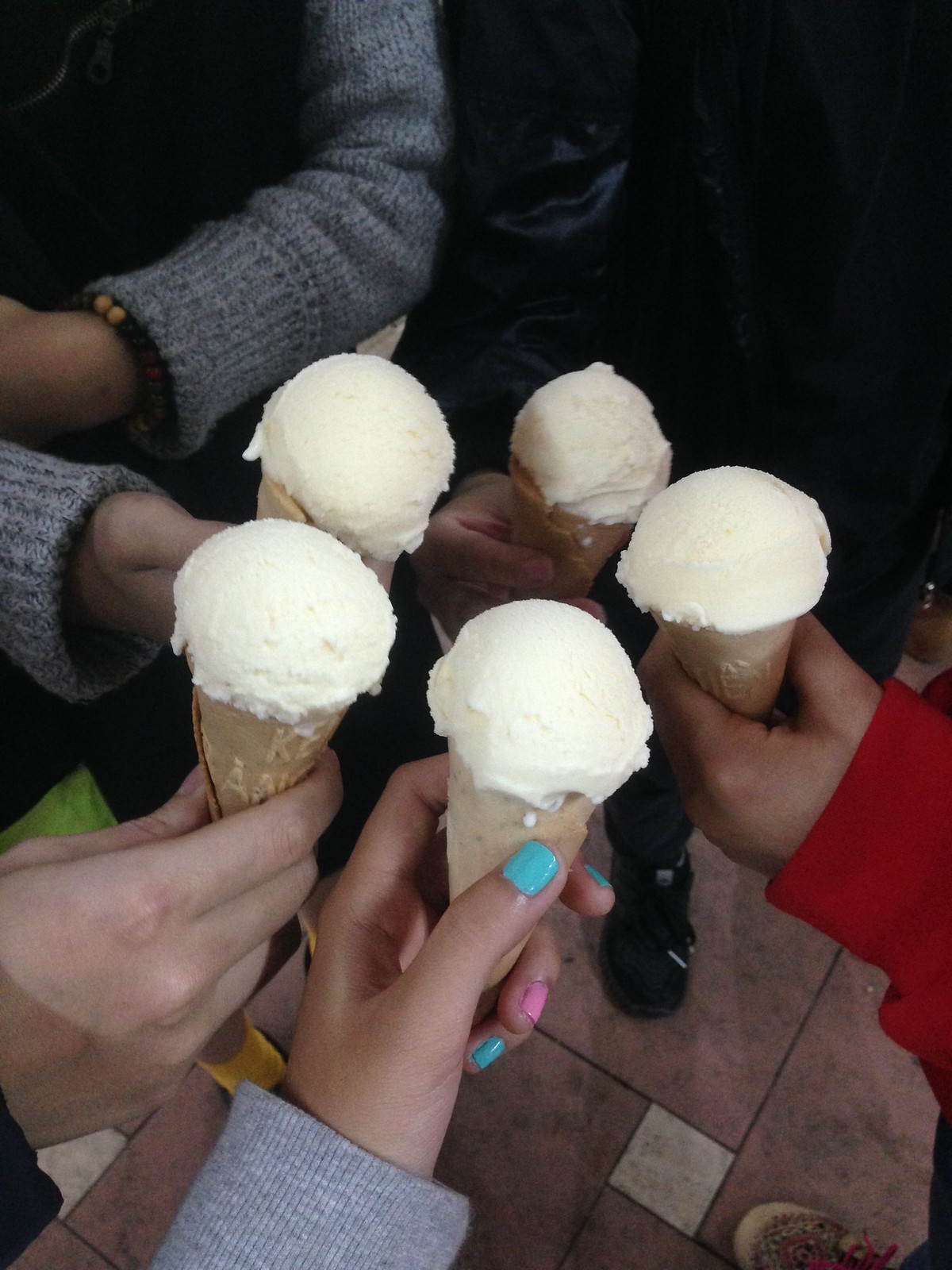In the photograph taken from overhead, five individuals are holding beige waffle-style ice cream cones topped with scoops of white vanilla ice cream, bringing them together in a toasting gesture. The focal point of the image is the five hands holding the cones, set against a red and white tiled floor. At the bottom, a hand with teal and pink painted nails holds a cone. Moving around clockwise, at about 7 o'clock, a hand with a cone emerges from someone in a gray sweater. At 12:30, a hand owned by an individual wearing a black leather jacket joins in. Another hand wearing a red shirt appears around 4 o'clock. The final hand completes the circle at about 5 o'clock. Although you can see parts of their outfits—such as a long-sleeved gray sweater, a red sweatshirt, and a black leather coat—the emphasis is on the communal and celebratory lifting of their uniform ice cream cones, symbolic of togetherness and shared joy.